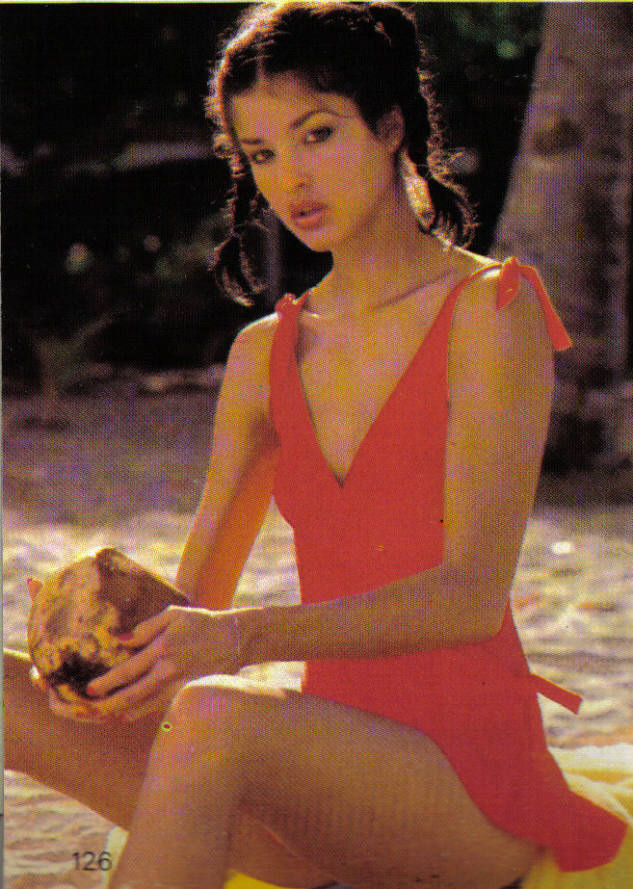This photograph depicts a young woman with dark black, braided hair, and a slender, angular face adorned with subtle makeup. She is seated on a beach, wearing a red one-piece bathing suit with a V-neck, a ruffled skirt, and ties on her shoulders. The overall aesthetic of the photo appears both old and grainy, giving it a vintage feel. The woman's expression is serious, with her mouth slightly open, perhaps suggesting an attempt to look seductive. 

She sits on a yellow towel with her knees up and elbows bent, holding a large beige seashell or rock. The background features beige sand, the base of a palm tree trunk over her right shoulder, and a mix of tropical foliage and blurred greenery over her left shoulder. The image captures her looking directly at the camera while seated on the sand, adding to the sense of candid intimacy. Below her, the number "126" is visible, adding another layer of detail to the scene.